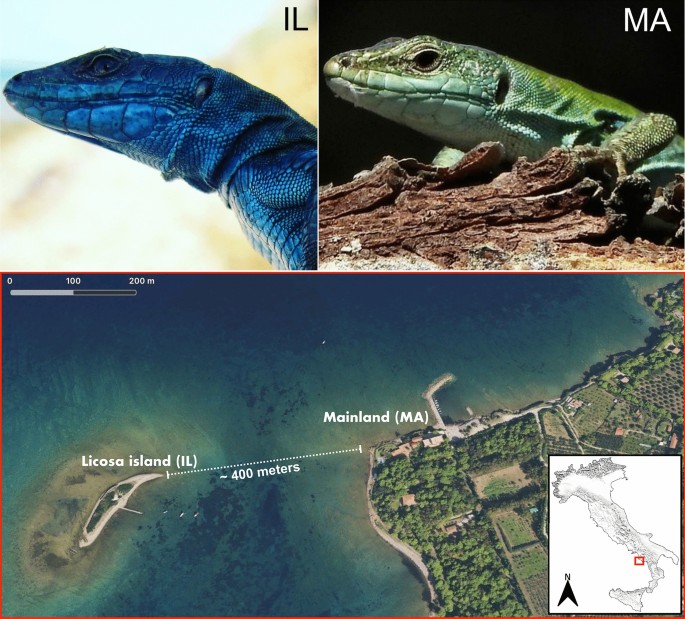This image is arranged in a slight horizontal rectangle, just a bit wider than it is tall, with three primary images. The top row features two side-by-side images of lizards. The left image depicts a blue lizard set against a gray background, labeled with the text "IL" in black font. The right image shows a green lizard on a piece of wood against a black background, with the text "MA" in white font.

Below these, the bottom image is a top-down aerial photograph taken from a couple of hundred feet in the air. It portrays La Cosa Island labeled with white text on the left, and "mainland MA" on the right, separated by a body of water, indicated by a dotted line. The image includes a scale from 0 to 200 meters in the top-left corner and depicts trees and land on the mainland, with minimal foliage on the island itself. In the bottom right corner of this image, there is an inset hand-drawn or sketched map of Italy in black and white. A small red box highlights an area on the west coast of Italy, and a black arrow with the letter "N" indicates the north direction.